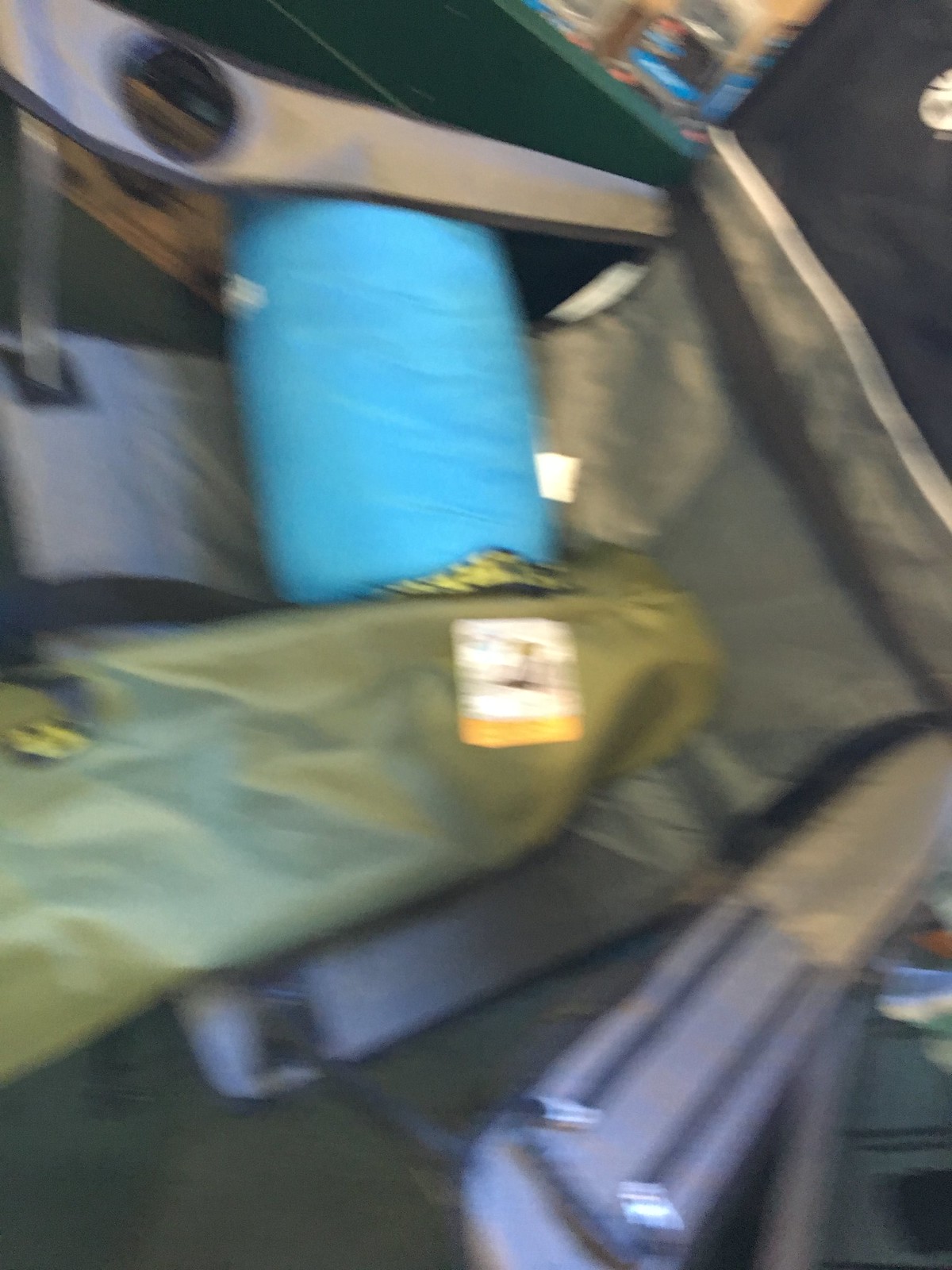In this slightly blurred image, a camping chair takes center stage. The chair, designed for outdoor use, features two armrests both shaded in blue. Prominently, the right armrest, located at the top left corner of the image, includes a built-in cup holder. Resting on the seat of the chair, there's a green item accompanied by a small, oblong blue item, which appears to be a pillow. The backrest of the chair is gray, transitioning into a striking design at the very top where a white line separates the gray from the blue background, adding a touch of color to its sturdy construction.